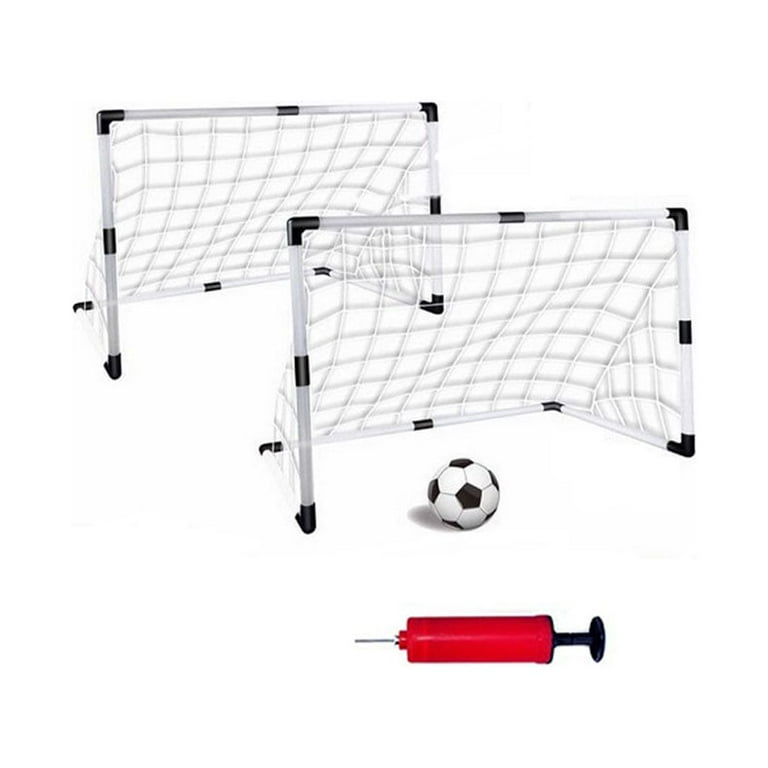The image features a stark white background that extends beyond the frame, creating an infinite white space. Centrally positioned are two large soccer goals, one positioned directly behind the other. Both goals are constructed with white piping and feature black corners and joints. The nets are predominantly white with a slight gray tint.

In front of the nearer goal sits a classic black and white soccer ball, positioned precisely at the center. Directly below the soccer ball, pointing toward the nine o'clock position, is a red ball pump with a black handle. The needle of the pump is prominently visible.

The composition is symmetrical and uncluttered, highlighting the clean, bright nature of the white background, making the colors of the soccer ball and pump stand out vividly.